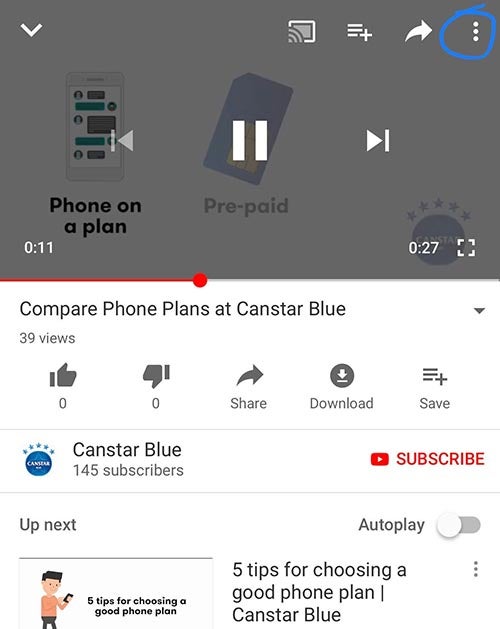This is a screenshot of an app featuring content from the CanStarBlue YouTube channel. At the top left of the screen, there's a faint gray-shaded drop-down arrow. Moving to the right, there's a Wi-Fi icon, followed by three horizontal lines next to an addition symbol, and a right-facing arrow. A cluster of three vertical dots circled in blue is also seen.

Centralized on the screen are media control buttons: reverse, pause, and fast-forward. The video progress bar indicates that 11 seconds of a 27-second video have elapsed. Below this, a caption reads, "Compare phone plans at CanStarBlue," with the video having amassed 39 views.

Action icons for thumbs up, thumbs down, sharing, downloading, and saving the video are visible. The channel name, "CanStarBlue," along with its subscriber count of 145, appears next to a prominent Subscribe button.

Directly underneath, a section labeled "Up next" features a thumbnail of a cartoon character—a male holding a smartphone in his left hand. This thumbnail advertises a video titled "Five Tips for Choosing a Good Phone Plan."